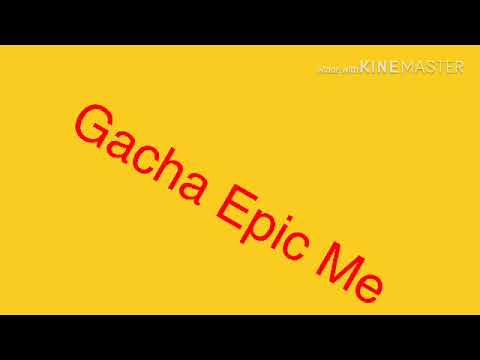This horizontally aligned rectangular image features thick black bars at the very top and bottom, enclosing a solid bright yellow background. Dominating the image, a diagonal red text slants from the upper left corner to the lower right corner, spelling out "GACHA EPIC ME" in all capital letters. In the upper right-hand corner, in small white text, is the phrase "MADE WITH KINEMASTER," with "KINEMASTER" in capital letters. The letters, both red and white, appear hazy and indistinct, possibly due to JPEG artifacting, creating a slight film grain effect on the image.